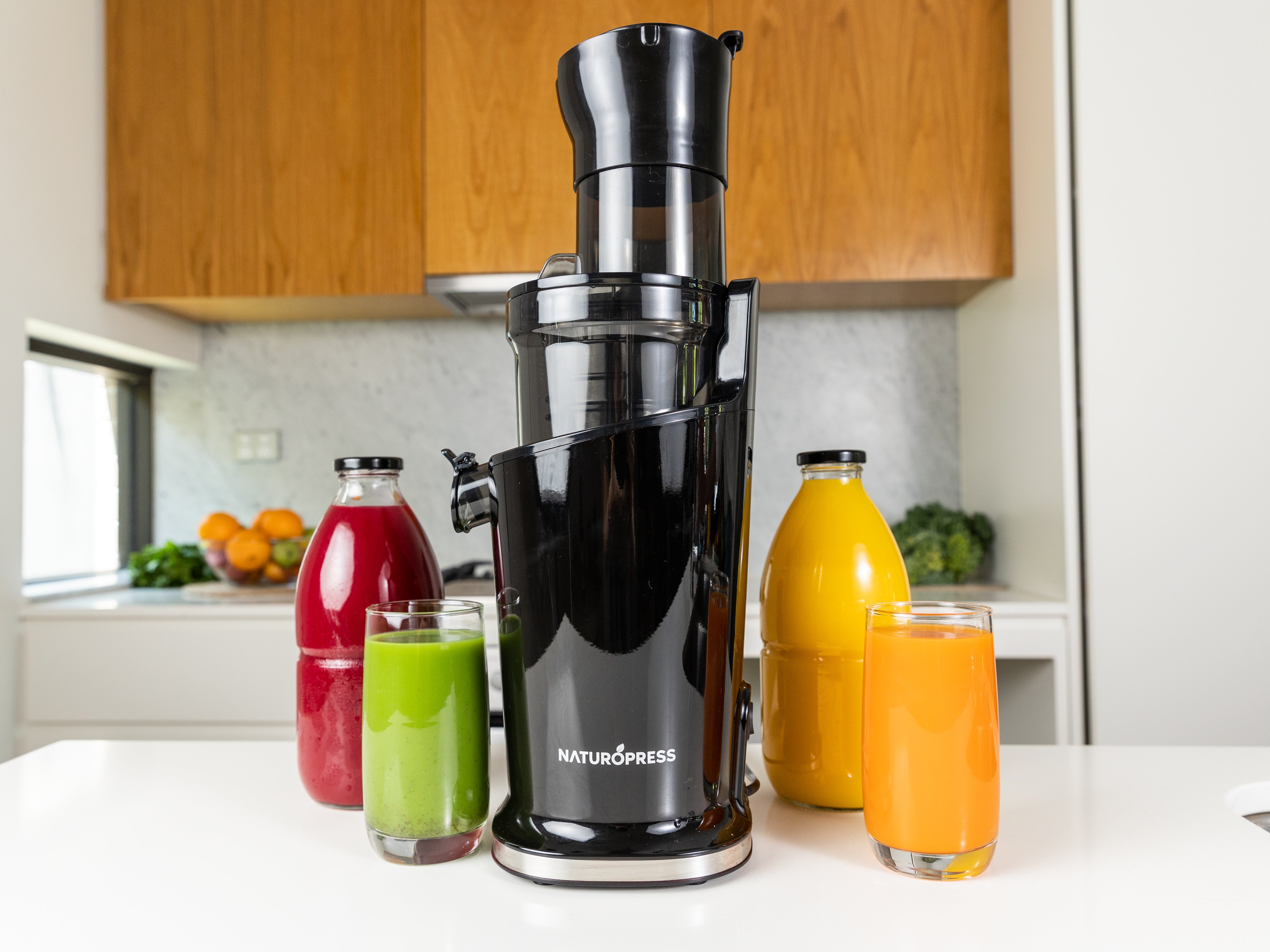On a sleek, white countertop stands a prominent black juicer labeled "Naturopress," approximately 18 inches tall. This sophisticated appliance features a top compartment for inserting fruits and vegetables, with a spout on the left side where juice is dispensed after the pulp is extracted. To the left of the juicer is a glass filled with green juice, accompanied by a bottle containing red juice behind it. On the right, a bottle of orange juice with a black cap sits beside a glass filled with the same orange liquid. The background reveals brown cabinets mounted on a wall and a gray-white mixed backsplash. The countertop behind the main scene is adorned with a variety of oranges and green vegetables, adding a touch of vibrant, fresh produce to the setting.